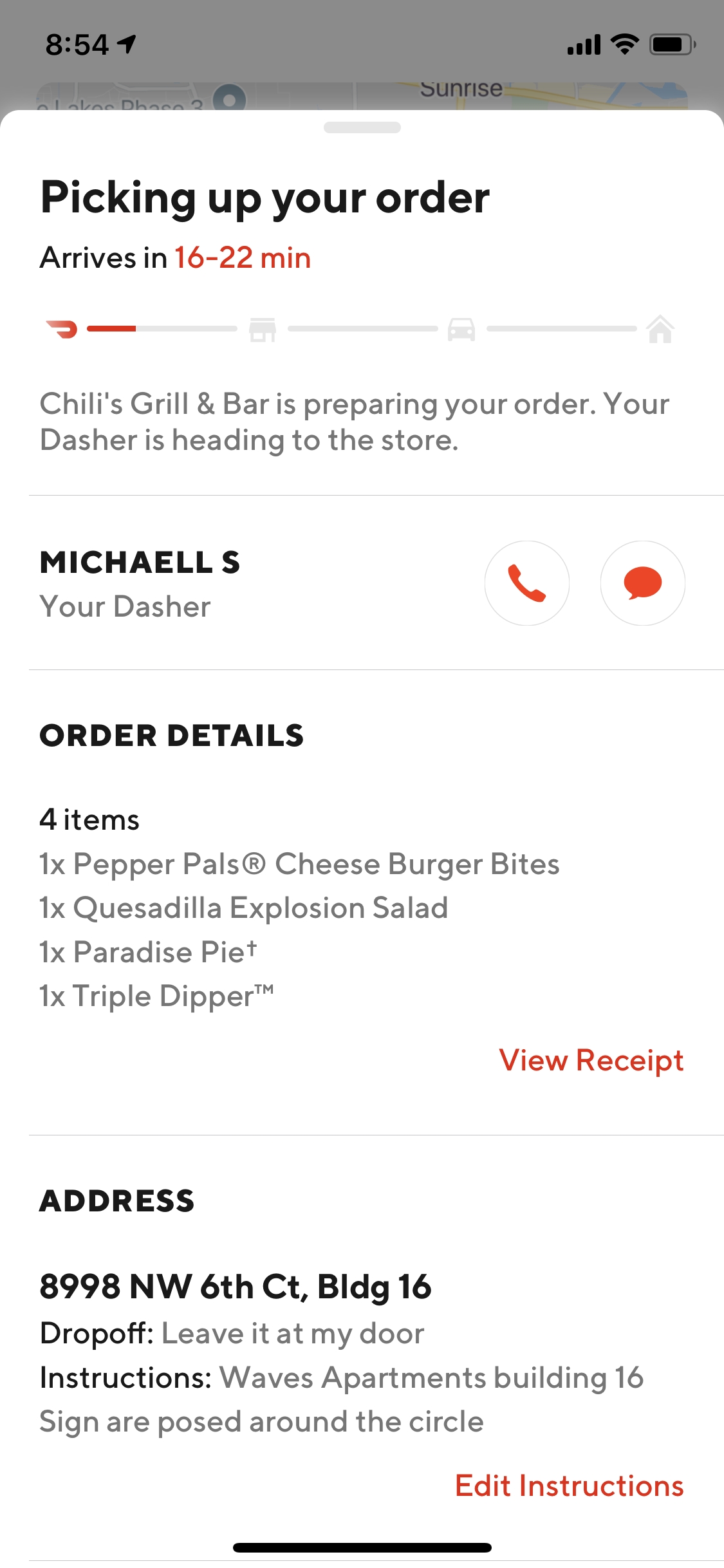The image displays a DoorDash order tracking screen. At the top, bold black text reads "Picking up your order," followed by smaller text indicating an estimated arrival time of "16 to 22 minutes" in red. Below this, a progress bar with four steps is visible, with the first step highlighted in red and featuring the DoorDash icon, while the remaining steps are in gray. 

The section below the progress bar states "Chili's Bar and Grill is preparing your order," and indicates that "Your dasher is heading to the store." A line divider separates this information from the details about the dasher. 

Next, it introduces "Michael, your dasher," with options to call or text him represented by red circular icons on the right. 

Further below, the screen is divided into two sections: "Order Details" and "Address," presumably detailing the specific order items and delivery location respectively.